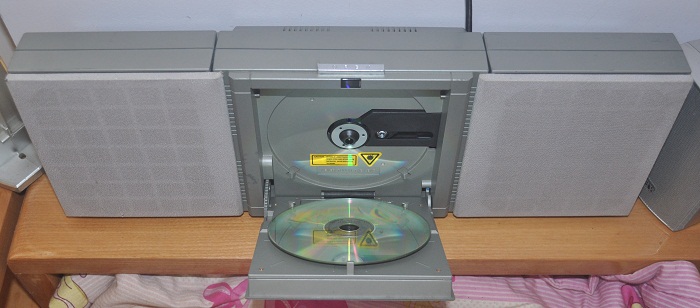This detailed photograph captures an old-style, silverish-grey boombox, taken from a slightly elevated angle. The boombox, with its two integrated speakers on either side, features a front-facing CD-ROM case that is open, revealing a CD without any identifiable title. The device, which can play one CD at a time, is designed so that the CD is mounted horizontally in a door that flops down for easy loading. A warning triangle likely indicating caution against disassembly is also visible. The boombox is placed atop a small wooden bench or table, resting on what appears to be pinkish-white fabric from a bed below. The background includes a grey wall that is a shade lighter than the boombox itself. There is no text in the image.